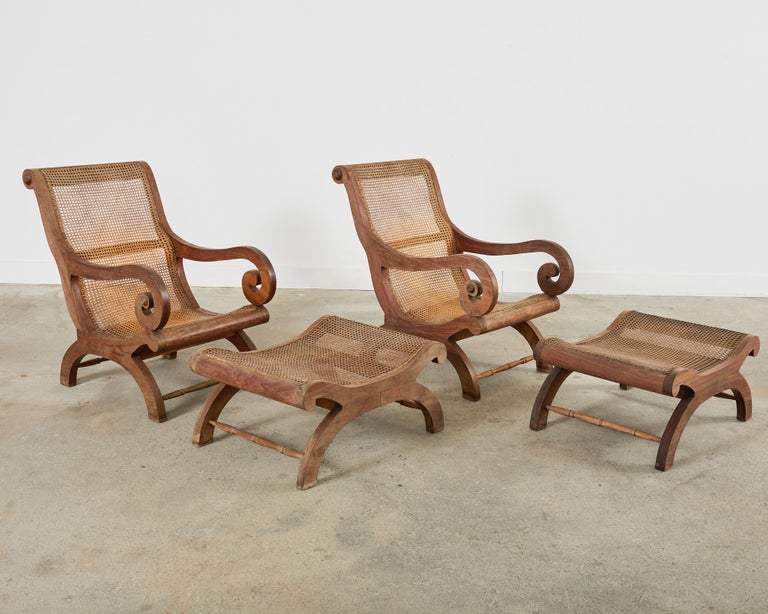The image showcases an indoor setting with a pair of matching wooden chairs accompanied by matching ottomans or footrests, all adorned with a see-through mesh cover. The chairs are designed with a low, laid-back, ergonomic slant, resembling a combination of Appalachian and handcrafted styles, featuring curved armrests that spiral at the ends and connect to arched bases supported by spindles. The ottomans mirror this construction with the same wooden arc and mesh design. The floor beneath these furniture pieces appears to be a grey, slightly stained cement or tile, and the backdrop is a plain, light cream or white wall, emphasizing the earthy tones of the brown and light orange furniture. The minimalist composition highlights the rustic yet elegant aesthetic of the set, free of any other objects in the image.